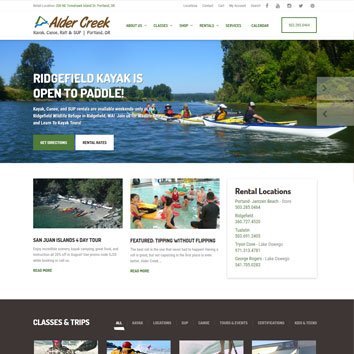This is a color image of a website. The overall image quality is very blurry, making much of the text difficult to decipher. At the top of the page, there is a partially legible logo that resembles a stylized drawing of a mountain. Next to the logo, the text "Alder Creek" is visible. Multiple menu items are present but are too blurry to read clearly. 

Below the header, there is an outdoor photograph depicting a tranquil lake scene. Several individuals are seen paddling kayaks on the calm waters. In the background, the shoreline is densely populated with trees, and the sky above is a clear, uninterrupted blue. Superimposed on this image, the text reads: "Ridgefield Kayak is open to paddle." Beneath this text, more writing is present but is too blurry to be legible.

Towards the bottom of the website, on the same photograph of the lake, there are two buttons: a green rectangle labeled "Get Directions" and a white rectangle labeled "Rental Rates." Further down, there is an overhead photograph of a building, but it is also too blurry to distinguish any details.

Adjacent to that, text reads "San Juan Islands and Bay Tour," accompanied by additional text that is too blurry to read. To the right of this, another photograph features a group of people in a pool. The accompanying text includes "Featured tipping without flipping," yet the details underneath are unreadable due to blurriness. Finally, the section labeled "Rental Locations" has more text below it that cannot be clearly made out.